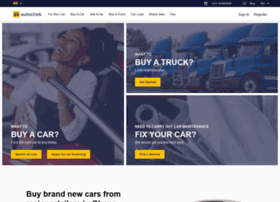The image is a low-resolution, blurry screenshot of a website, making the finer details difficult to discern. At the top of the screenshot, there's a black bar with some white text on it, though the specifics of the text are unclear. Just below this, there is a white bar featuring black text alongside a yellow icon on the right side.

The main body of the screenshot includes three distinct segments, each with an image and some accompanying text. Starting from the left:

1. **Left Segment:** The first image features a smiling Black woman looking up at the sky while holding a metal pipe. She is wearing a white top. Superimposed on this image in white font is the text: "Buy a car?"
   
2. **Middle Segment:** The second segment is divided into two images:
   - The top image shows four blue truck cabs lined up in a row. The text "Buy a truck" is superimposed over this image.
   - Below it, there's another image that appears to be of a ratchet tool, with the phrase "Fix your car?" overlaid in text.

3. **Right Segment:** Although less defined, there's a continuation of images following a similar style, but the specific contents are harder to identify due to the image quality.

All of these images seem to have a gray filter applied to them. Below these segments is another white bar with black text that reads: "Buy brand new cars from," but the continuation of this text is cut off by the edge of the screenshot.